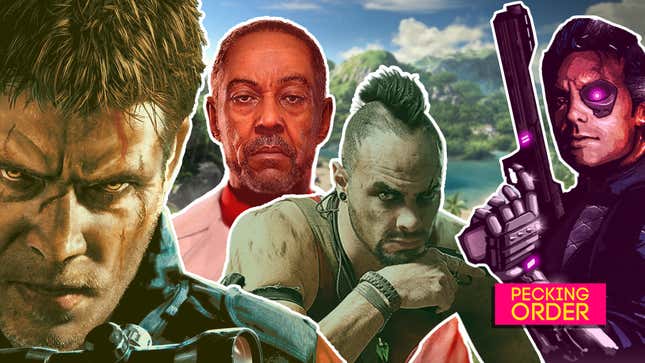In this vertically framed advertisement titled "Pecking Order," set against a scenic background of blue skies, fluffy clouds, mountain ranges, and lush vegetation, four distinct and vividly detailed warriors are depicted from left to right. The first man on the left has a light-skinned complexion with lighter-colored, perhaps blonde or light brown, hair and amber-colored eyes. His face is marred with scars and he wears a black vest, exuding an angry, aggressive demeanor. The scope of a weapon is visible near his chin.

Next to him is a stoic, dark-skinned man, identified as Giancarlo Esposito, who sports a neat mustache and beard. He wears a white jacket with a striking red collar and looks directly at the camera without expression. In front of Esposito stands a light-skinned man with an intimidating grimace, a prominent mohawk, and a goatee. He is adorned with various items including wristbands and bands around his biceps, suggesting a rugged and battle-ready nature.

The final figure on the right is a half-human, half-cyborg individual with a mechanical eye and arm. He is holding a purple gun with an extended barrel pointed upwards. One half of his face features a red, mechanical eye while the other half appears normal. The term "Pecking Order" is prominently displayed in a pink rectangular box with yellow text in the lower right-hand corner, emphasizing the hierarchical theme of the image.